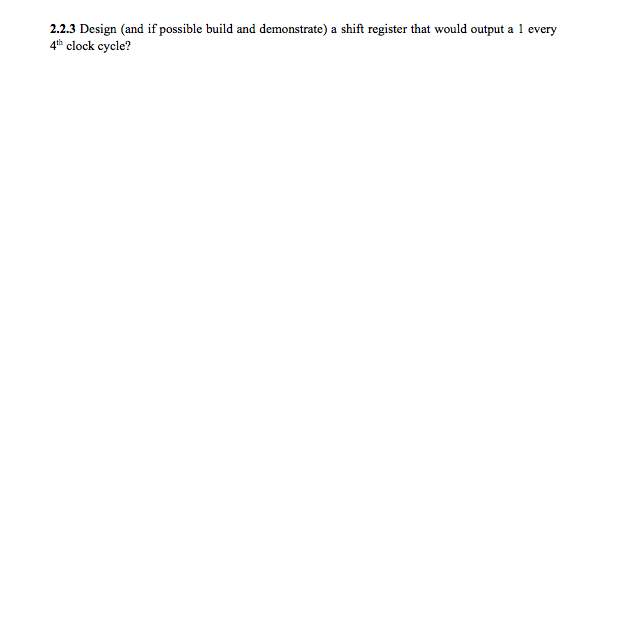The image displays a segment of text from a website. The text begins with the numeral "2.2.3" in a bold, black font. Adjacent to this, in a lighter, finer print, is the word "Design" with a capitalized "D". Following this, within parentheses, it reads: "(if possible, build and demonstrate)". The parentheses then close, and the text continues: "a shift register that would output a 1 every 4th clock cycle?" where the "1" and "4" are depicted as numerals, and "4th" includes a "th" superscript. The background of the page is entirely white.